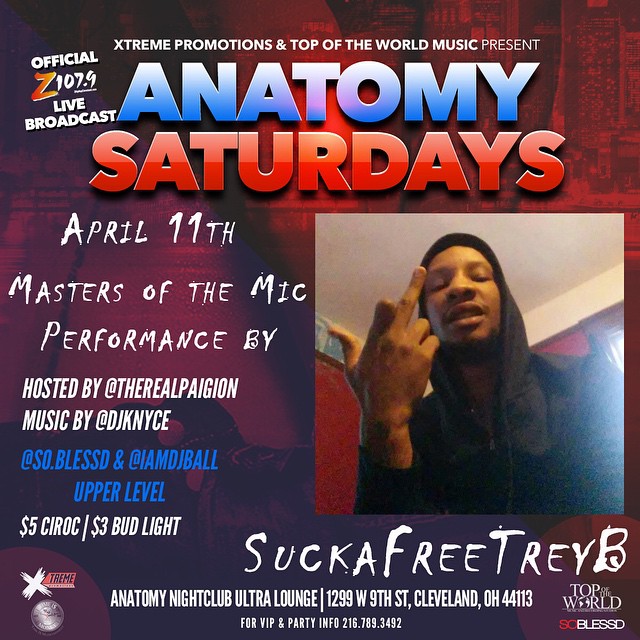The advertisement features an adult-oriented event at the Anatomy Nightclub Ultra Lounge, located at 1299 West 9th Street, Cleveland, Ohio, 44113, presented by Extreme Promotions and Top of the World Music. The central image depicts an African-American man in a black hoodie, photographed indoors, raising his hand with writing on it and flipping off the camera. The ad promotes "Anatomy Saturdays," highlighted in bold text, with "Anatomy" in blue and "Saturdays" in red, both written in capital letters. The text details an "Official Z107.9 Live Broadcast" set for April 11th. The event, branded as "Masters of the Mic," features a performance by "Sucker Free Trey Bae," hosted by "The Real Pageon," with music by DJs including "DJ KNYCE," "So.Blessed," and "IamJayBall." Drink specials include $5 Ciroc and $3 Bud Light. Additional event details emphasize that the club is an adult venue.